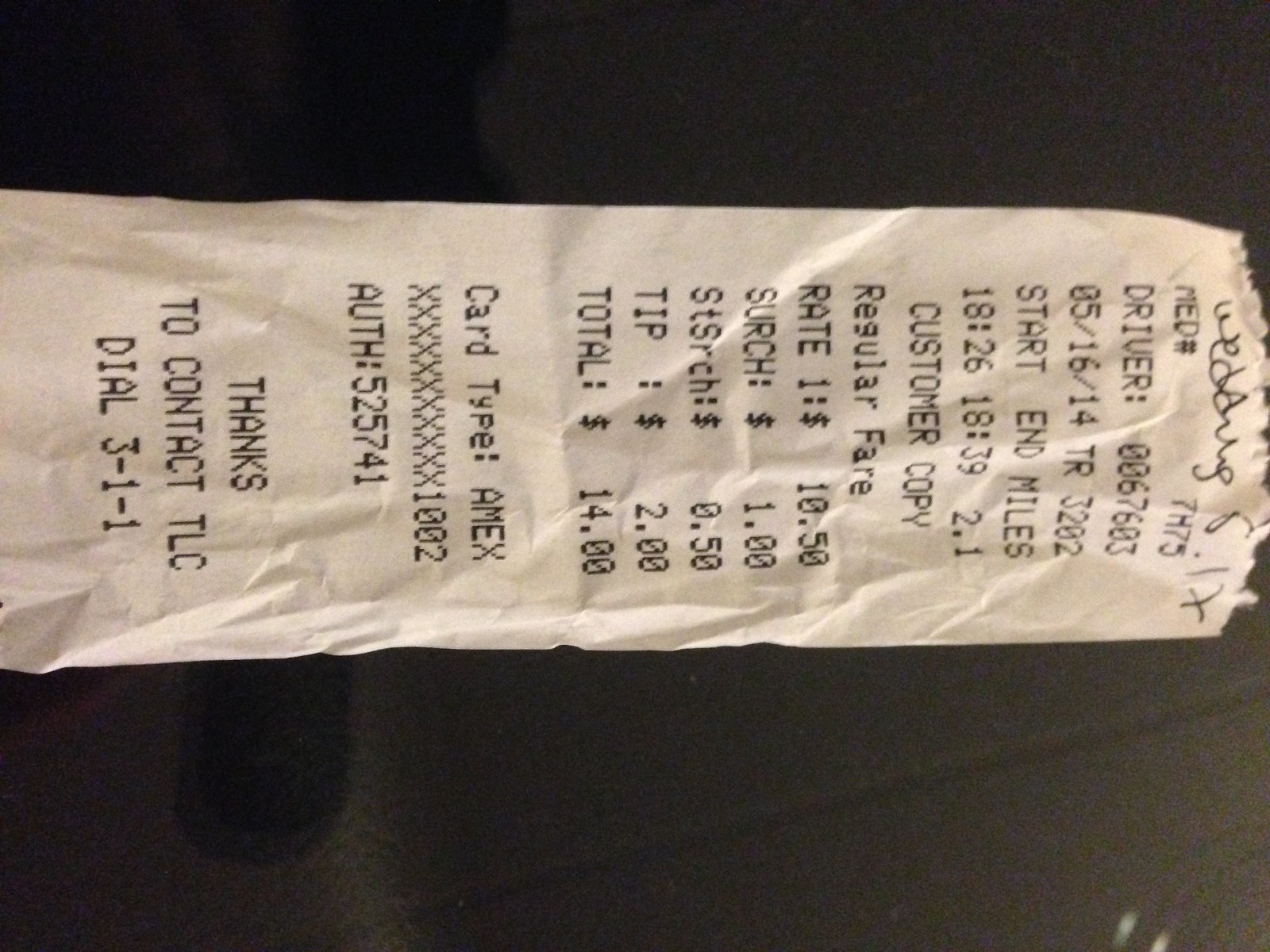This image depicts a white receipt with numerous lines of black text. At the top of the receipt, the driver identification number "0067603" is prominently displayed. Further down, the phrase "Customer Copy" is printed, indicating that this receipt is intended for the passenger's records. The regular fare rates are itemized, amounting to a total of $110.50. Payment was made using an American Express card, as denoted by "Card Type: Amex." At the bottom, there is a note encouraging customers to contact the Taxi and Limousine Commission (TLC) for any inquiries or feedback by dialing 3-1-1.